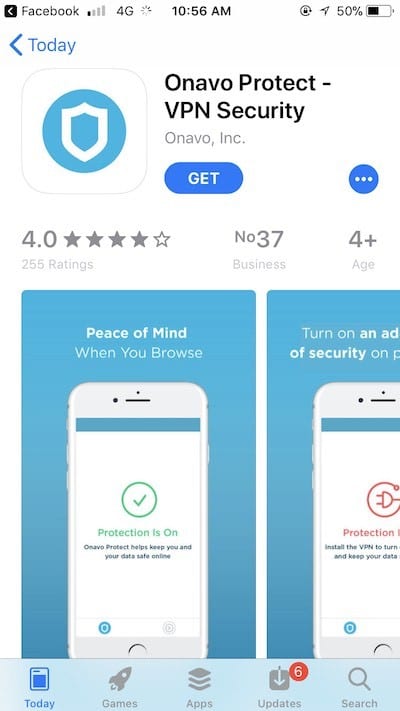This image is a vertical rectangular screenshot taken from a smartphone. The top section of the screen is the typical status bar seen on many devices, featuring the Facebook header in black text. To the right are indicators showing a 4G connection, the time as 10:56 AM, and the battery at 50%.

Below the status bar, the background is white. In the upper-left corner under the Facebook header, "Today" is written in turquoise text, accompanied by a left-pointing arrow. Directly underneath, in the middle, is another rectangular section with rounded corners and a white background. Centered in this section is a turquoise circle with a white shield inside it, symbolizing the Onavo Protect app.

Next to the shield icon, the text "ONAVO Protect" is in bold black, followed by "VPN Security" in all capital letters except for the "S." Below this headline appears "ONAVO, Inc." in light gray font. Further down, there is a bright blue, horizontally-oriented rectangular button with the text "Get" in lighter letters. Adjacent to it on the right is a smaller blue circle with three lighter-colored dots arranged vertically.

Further down the image, in gray font, is the rating: "4.0" with four out of five stars filled in. To the center, the text "No. 37" and to its right, "4+" indicating age compatibility. Beneath "No. 37," the word "Business" is written, and beneath "4+," it says "Age." There are 255 ratings listed in lighter font.

Two more vertical rectangular sections are located further down, each with a turquoise background. The first section's title is "Peace of mind" in bold text, followed by the phrase "when you browse" in non-bolded font. This section features an image of a smartphone with a white border around it and a turquoise stripe across its top. The center of the phone image has a white area with a green circle and a green checkmark, declaring "Protection is on" in green text with additional black text below.

The second section to the right is partly cut off by the image's edge. It contains text reading "Turn on an AD" and "of security on," but only part of these lines are visible. This section also displays half of a smartphone image where the text "Protection" in red and a symbol of a red circle with a plug is seen above it, followed by some additional text.

At the very bottom is a light blue horizontal bar with icons and corresponding labels: "Today," "Games," "Apps," "Updates," and "Search," for easy navigation.